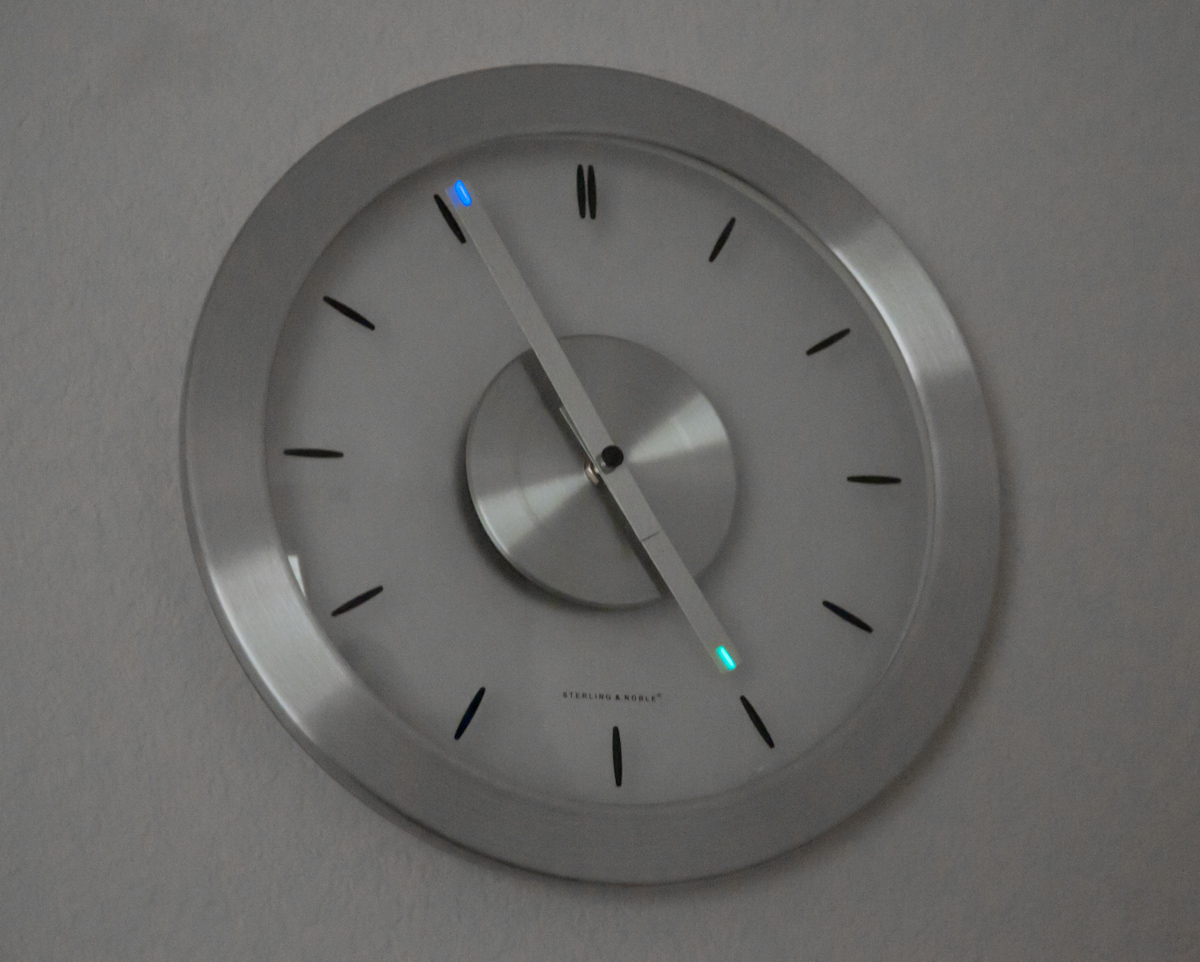The image features a large, high-tech digital clock mounted on a gray wall, with the clock positioned centrally in the frame. The clock has a sleek design with a silver disc at its center and a silver border around a glass number face. The numbers are represented by black tick marks. Enhancing its modern aesthetic, the clock uses colored lights: a blue light for the minute hand and a turquoise light for the hour hand. The hands on the clock show that the time is approximately 5:56 p.m. Beneath the clock's center, there is a small label that reads "Sterling R. Noble." The predominant colors in the image are blue, teal, silver, and black, lending the clock a sophisticated and contemporary appearance suitable for an office or home setting. The lighting creates a subtle sheen on the clock, adding to its modern look.